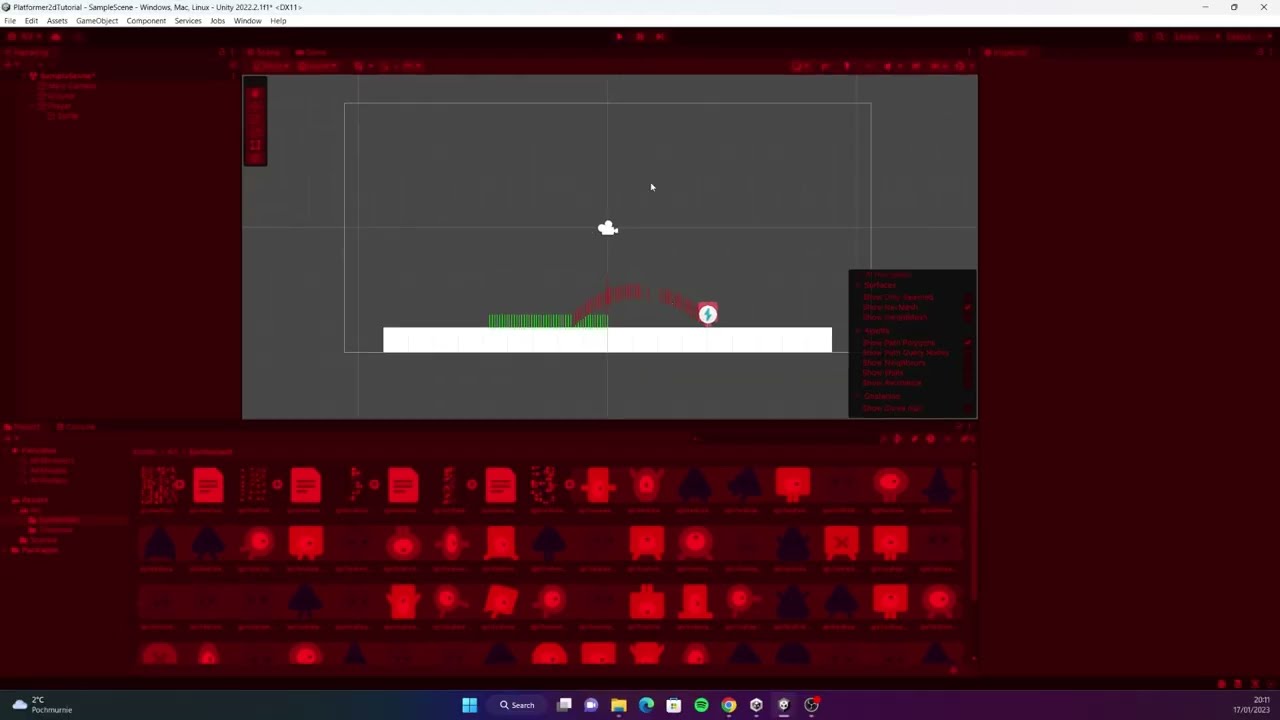This image depicts a computer screen displaying an indistinct application with numerous intricate details. At the top, there is a thin horizontal gray bar featuring conventional menu options such as "File" and "Edit," along with window control buttons, including a closeout 'X' in the upper right corner. 

The center of the screen showcases a gray box with a mix of green and red lines, and symbols including a video camera emoji and a lightning bolt-shaped figure. There’s a gray horizontal rectangle with white lines below this. 

The background is primarily a dark, blood-red hue, adding a layer of complexity to the visual. The lower part of the image contains a horizontal bar indicative of a typical computer desktop interface, displaying various colorful icons like Google Chrome, Firefox, Spotify, and more, alongside a weather notification indicating it’s 2 degrees Celsius, accompanied by a white cloud symbol. 

This photograph or screen capture reflects a rather confusing yet detailed layout, possibly from a specialized program, the purpose of which is not entirely clear.